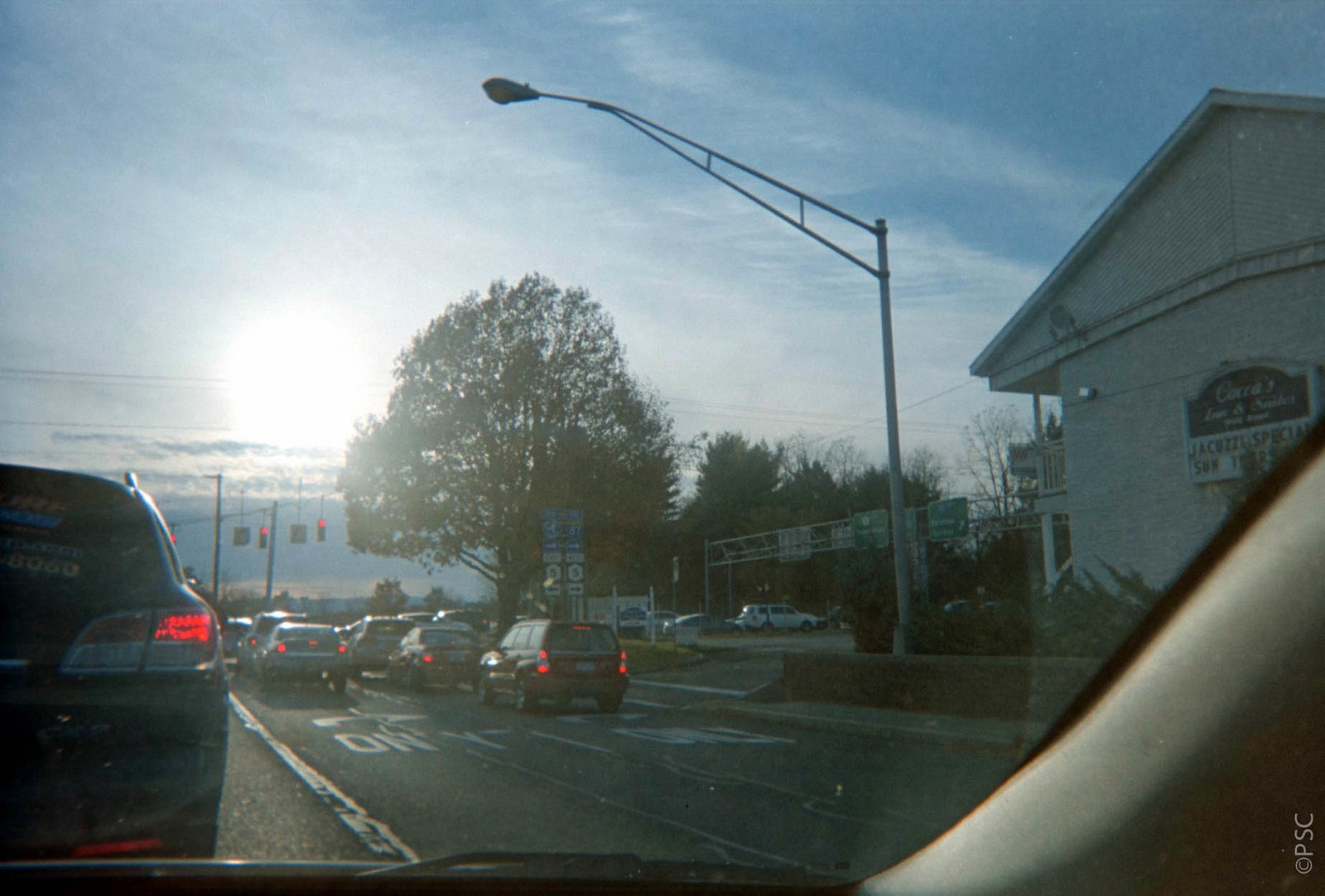From the perspective of a car's right-hand passenger seat at a traffic stop, the scene ahead depicts a busy intersection in New York State. The traffic light up ahead shines red, halting the cars in the lane designated for either straight travel or left turns. To our right, two lanes are clearly marked for right turns only. Adjacent to the intersection stands a white building featuring an illuminated sign. While the top portion of the sign is difficult to decipher due to its dark, scripted font, the movable letters below advertise a "Jacuzzi Special Sunday." Overhead, a New York route sign and another indicating junction with Route 81 confirm our location within the state's road network.